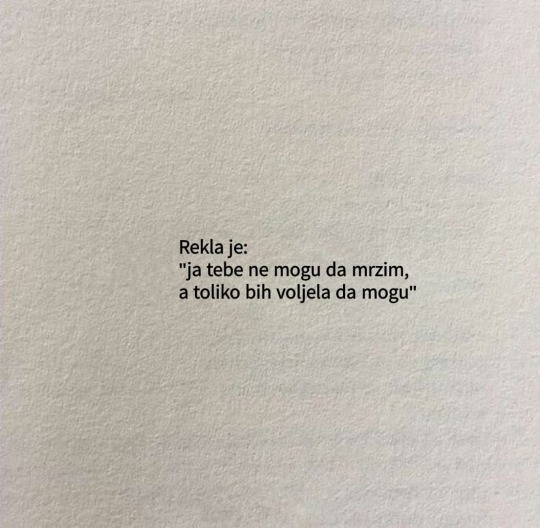The image is a detailed close-up photograph of a book page, showcasing a section of text printed in small black font on a creamy white background, possibly with a slight texture indicating paper fibers. This text is centered on the page and appears to be a quote or a short poem in a foreign language. It reads: "Reclaje;; 'Jatembe namungu da maraz, toklio ba volja da mungu.'" There are no other objects or colors visible in the image, just the text in the middle of an otherwise blank page, giving an impression of simplicity and focus on the words themselves. The precise language and meaning of the text remain unclear.